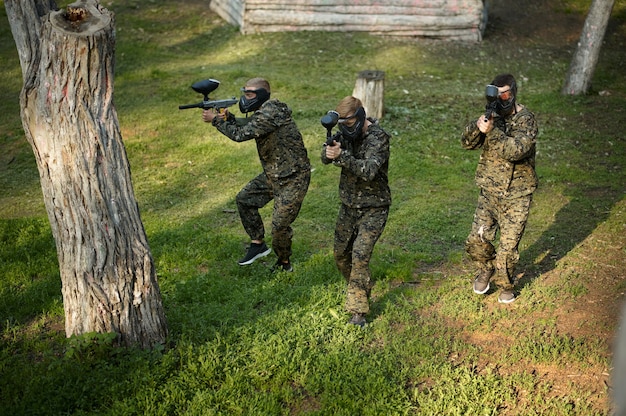This photograph showcases three determined men actively engaged in a paintball match, dressed head-to-toe in camouflage attire. Their faces are obscured by black paintball masks featuring goggles with orange-tinted lenses and protective mouth covers. The men, two with short blonde hair and one with short brown hair, are positioned in a tactical V-formation, cautiously advancing through a grassy and partially bare field. Each wields a black paintball gun equipped with a distinctive, football-shaped hopper. 

The surrounding environment includes a mix of light grass and bare patches of dirt, indicating sporadic ground cover. A prominent tree trunk occupies the left side of the image, while several tall, cut stumps and additional trees are visible in the background. These remnants of trees cast dappled shadows, suggesting the scene is lit by the afternoon sun. Behind the men, wooden structures crafted from horizontally stacked logs serve as barricades, further reinforcing the paintball park setting. The men each wear standard sports shoes — two in black and one in brown — as they navigate the challenging landscape.